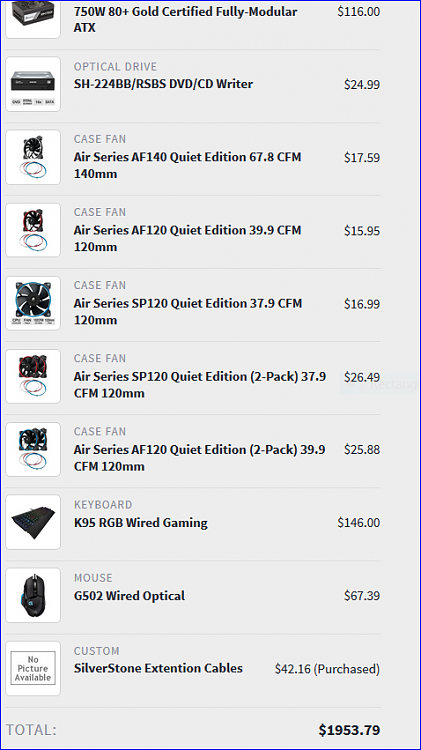The image showcases a variety of high-end components and peripherals for a custom-built computer, all neatly arranged within their respective boxes. 

1. **Power Supply**: The centerpiece is a 750W 80 Plus Gold Certified Fully Modular ATX power supply, priced at $116.
2. **Optical Drive**: Directly beneath the power supply is a DVD/CD writer, encased in a black box, valued at $24.99.
3. **Case Fans**:
    - Air Series AF140 Quiet Edition for $17.59.
    - Another case fan priced at $15.95.
    - A Quiet Edition case fan for $16.99.
    - Two additional case fans: one for $26.49 and the other for $25.88.
4. **Keyboard**: The K95 RGB Wired Gaming Keyboard, priced at $146, is situated below the case fans.
5. **Mouse**: A G502 Wired Optical Mouse, costing $67.39, is placed below the keyboard.
6. **Extension Cables**: Custom Silverstone extension cables at $42.16.

The combined cost of these components totals $1,953.79.